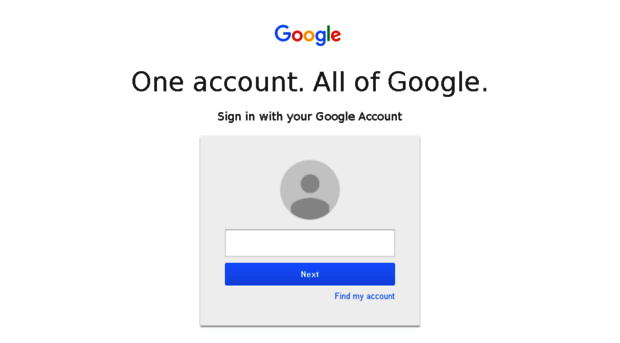The image depicts a Google sign-in screen without a border, featuring the iconic Google logo prominently at the center. The logo spells "Google" with the following color scheme: a blue capital G, a red O, an orangey-yellow O, another blue G, a green L, and a red E. 

Above the logo, in bold black font, the text reads: "One account. All of Google." Directly below this is another line of text in smaller black font centered within the image, stating: "Sign in with your Google account."

Beneath this text is a gray box containing a generic profile picture icon—a simple gray silhouette of a person. Accompanying this box is a field for entering login credentials.

Below the input box is a long rectangular blue button. Centered on the button in white text, likely in a font size of 8 or 10, is the word "Next" with a capital N.

Positioned to the very right end of the blue button is a hyperlink titled "Find my account."